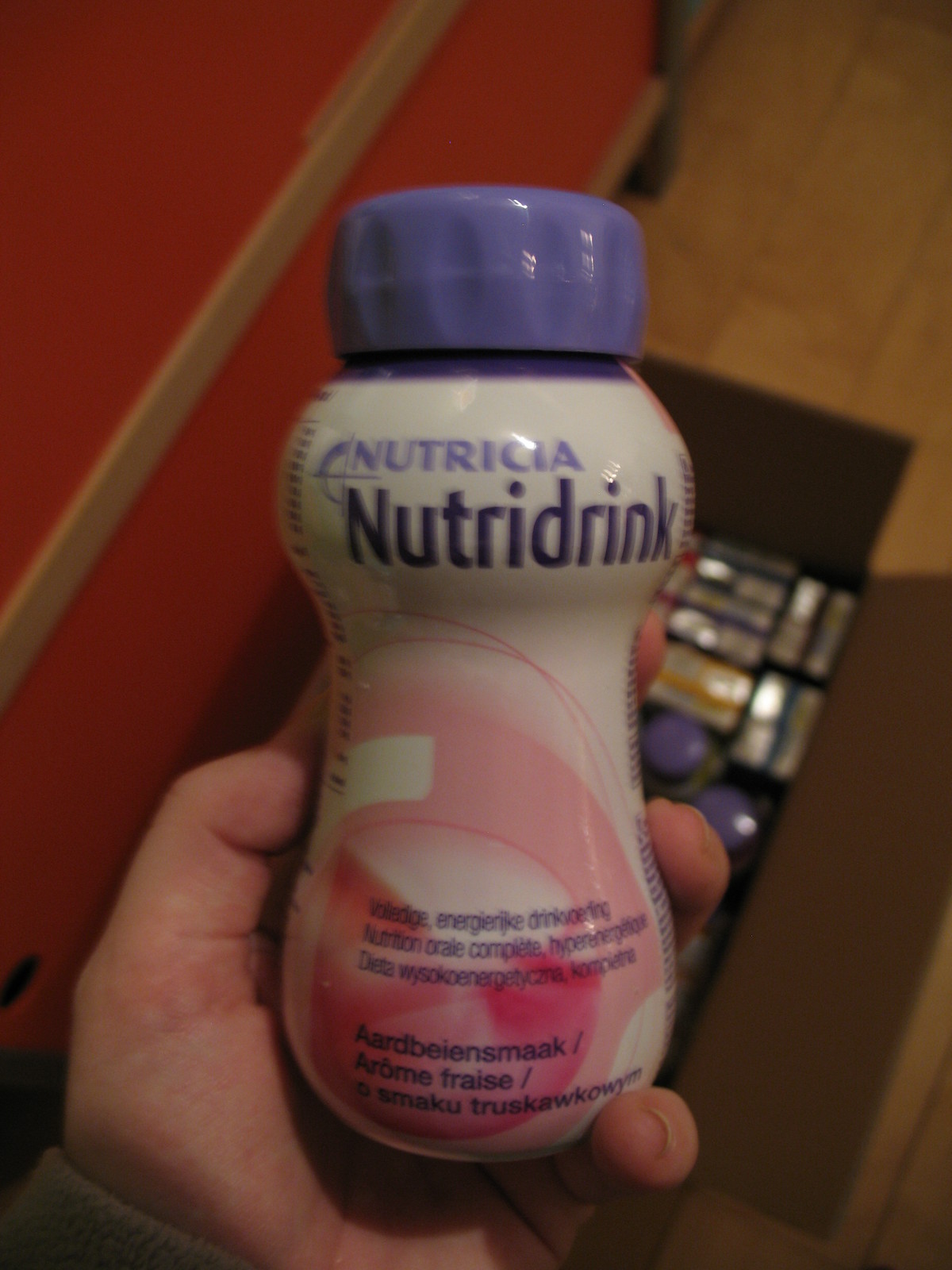This photograph, though slightly blurry, captures a scene from an overhead perspective. It reveals a wooden floor and what appears to be a shop cabinet or wall in the background. On the floor, there is a box filled with various items. The person's left hand is prominently holding a bottle labeled "Nutricia Nutri Drink." The text on the bottle primarily appears in a language other than English, but it clearly displays the flavor as strawberry. The bottle features a white label with pink accents and a purple lid.